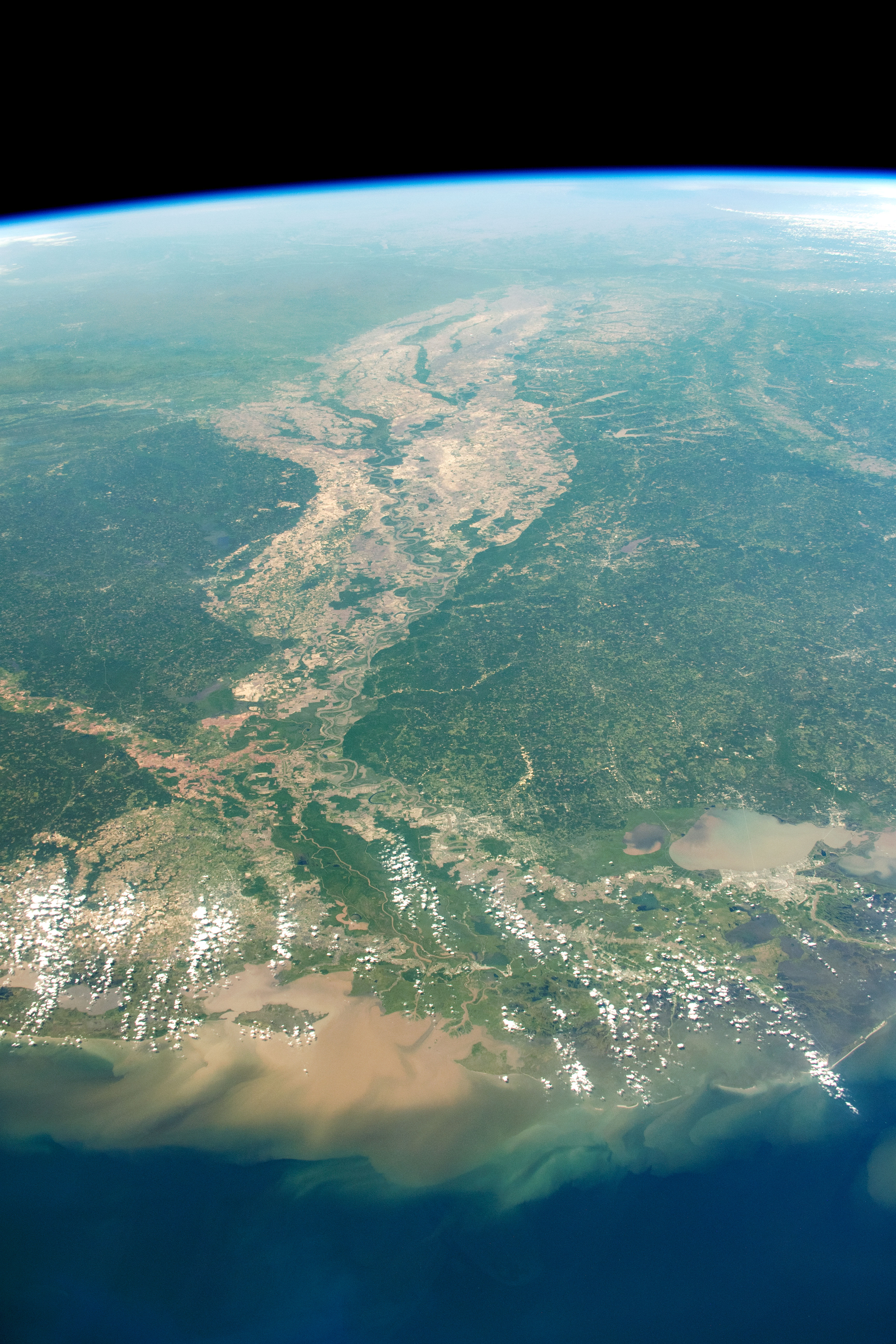This captivating outer atmosphere photo showcases a segment of Earth against the black backdrop of space at the top. The curvature of the Earth is highlighted in an electric blue hue that seamlessly transitions to the medium blue of the ocean below. The shoreline is defined by a stretch of tan sand. The landscape is predominantly green, representing forested areas and the tops of trees, interspersed with brown trails and cleared spaces that dot the terrain. Wispy clouds float over this vibrant scene, adding to the ethereal beauty of the photograph. The entire color palette of the image is dominated by shades of blue, with touches of green and tan, creating a serene and captivating view from space.